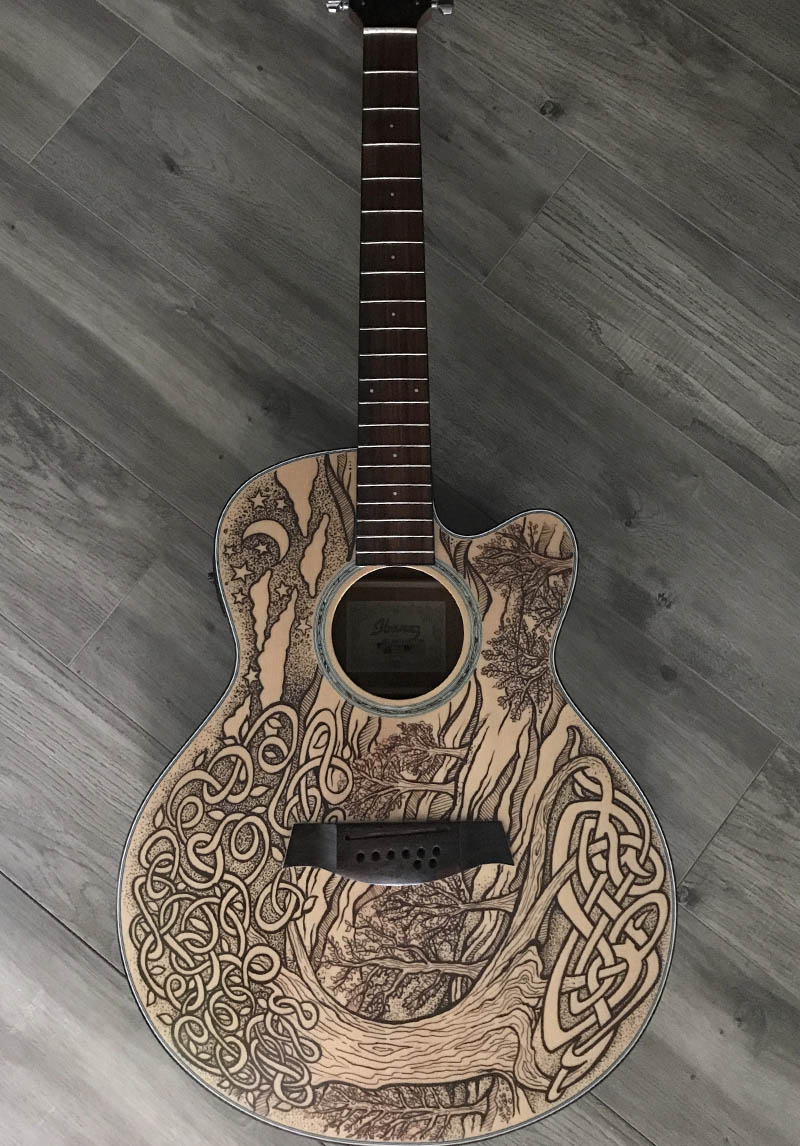This is a detailed photograph showcasing a custom-made acoustic guitar with an intricate and elaborate design. The guitar, displayed on a deep gray, wood-textured floor, is devoid of strings, suggesting it may still be in the process of being made. The neck of the guitar is a rich brown color and features silver frets. The front face of the guitar is a captivating canvas of artistry, rendered through a scrimshaw-like method involving dark and light coloration. Central to the design is a prominently carved tree with its sprawling roots entwined in a Celtic knot pattern. The limbs of this tree wind and intertwine up both sides of the guitar's body, forming complex, snake-like curves. Complementing this central motif are additional trees etched into the wood, creating a forest-like scene. In the upper part of the guitar, the design transitions to a serene sky scene featuring clouds, a quarter moon, and stars, adding depth and celestial charm to the artwork. Despite the absence of strings, the guitar appears to be structured for six strings, with a horizontal black piece where the strings would traditionally be affixed.